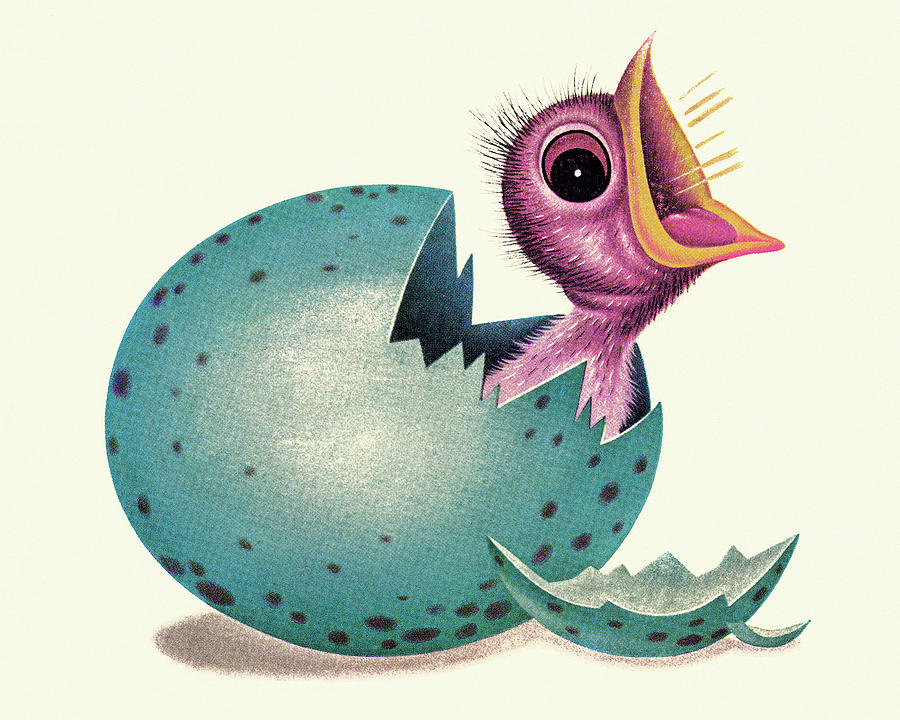The image is a detailed color illustration set against a pale, yellowish ivory background. It features a large, cracked, turquoise blue egg adorned with scattered dark polka dots, resting on a shadowed surface. Emerging from the broken shell is the profile of a fuzzy, purple baby bird, with a wide open, expressive eye and a red tongue visible inside its gold, open beak. Golden lines radiate from the bird's mouth, suggesting it's making noise. The bird's head and part of its neck are visible, covered with short, stiff black strands, indicating the sprouting of new feathers. A sharp, jagged piece of the eggshell is lying in front of the egg, enhancing the sense of the bird just hatching. The illustration uses vibrant purples and blues against the subtle background to highlight the newly hatched chick's startling and noisy emergence.